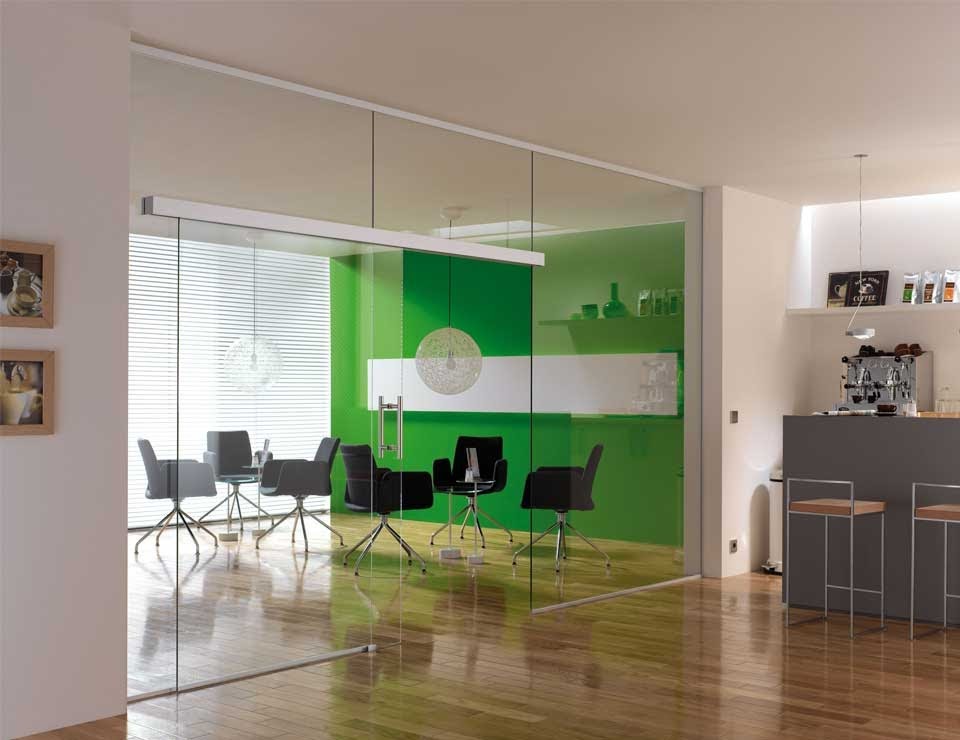The image shows a well-appointed break room within an office space, marked by its polished hardwood floors that reflect light. On the right side, there is a counter equipped with a stainless steel espresso machine and a few stools for seating. Above the counter, a white shelf holds packets of coffee, accompanied by a sign that reads "coffee."

Adjacent to this space, separated by floor-to-ceiling glass walls, is another room. This inner room features a bright green wall and a window that provides a view to the outside. The room contains two groups of three black office chairs, possibly arranged for meetings or discussions. Additional details include a couple of photographs on the wall to the left and what appears to be a white screen or piece of art on the green wall. The entire area, both the break room and the inner room, shares the same gleaming hardwood floor that enhances the sophisticated atmosphere.